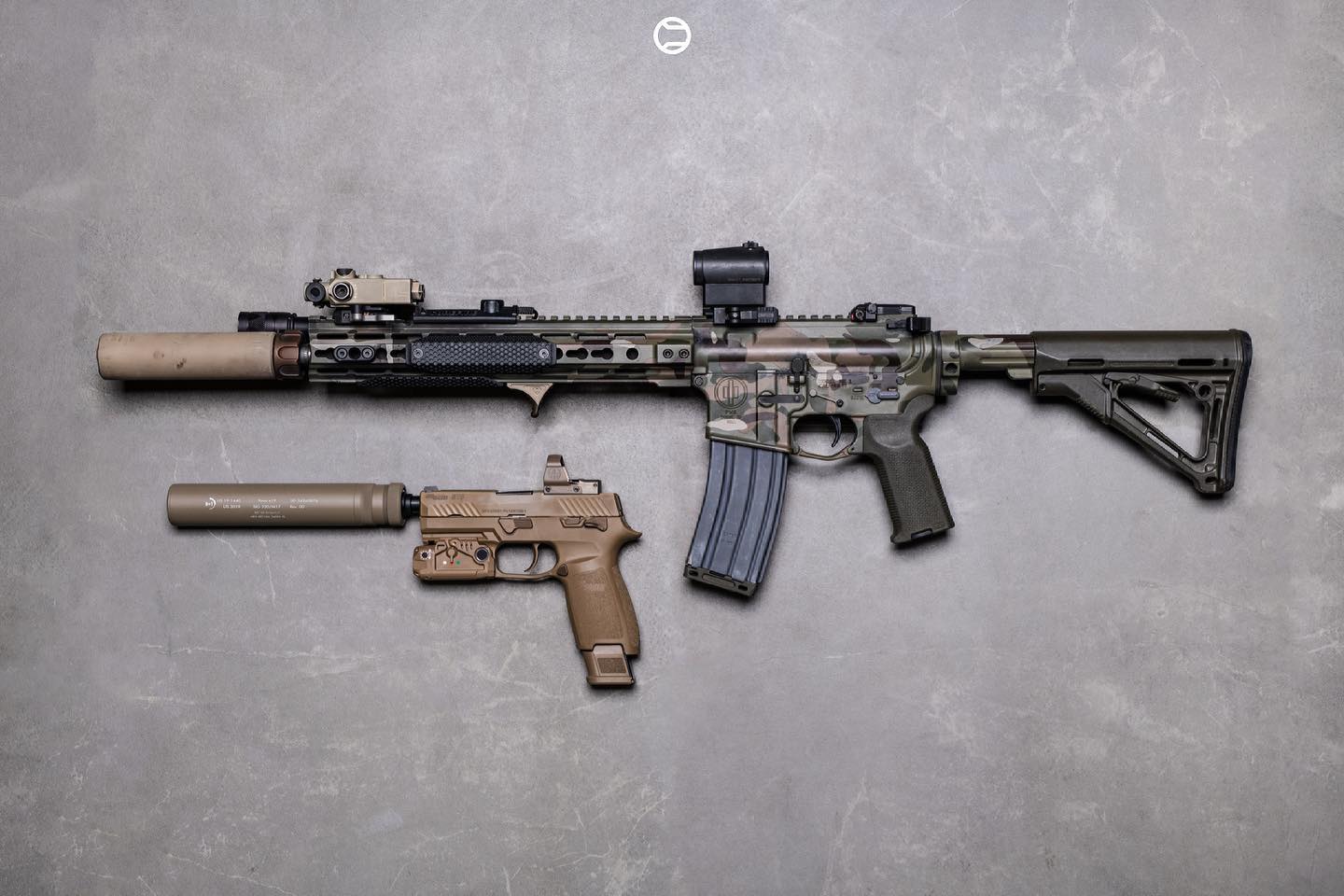This photograph captures two firearms set against a gray mottled surface that resembles stone or concrete. The larger firearm, an AR-15 rifle, is predominantly black with brown and gray components, featuring a combination of a black handle, a protruding black magazine, and a brown gun handle. It has a long barrel that narrows to a cylindrical tip, complete with a sight at its end and a black scope mounted on top. The rifle's body presents a green camouflage pattern, adding a realistic touch. The second, smaller firearm is a brown automatic pistol, possibly a Colt slide-action, equipped with a darker brown cylindrical silencer attached to its short barrel. This pistol also has a lighter brown hand grip and an extended magazine. The detailed surface on which these guns rest includes an irregular white pattern, reminiscent of scratches, and a small round logo with two curved lines at the center top, devoid of any writing. The overall aesthetic and arrangement evoke a scene that could be from an action movie, with the weapons' colors and design offering a potential blend between realistic and cinematic appearances.